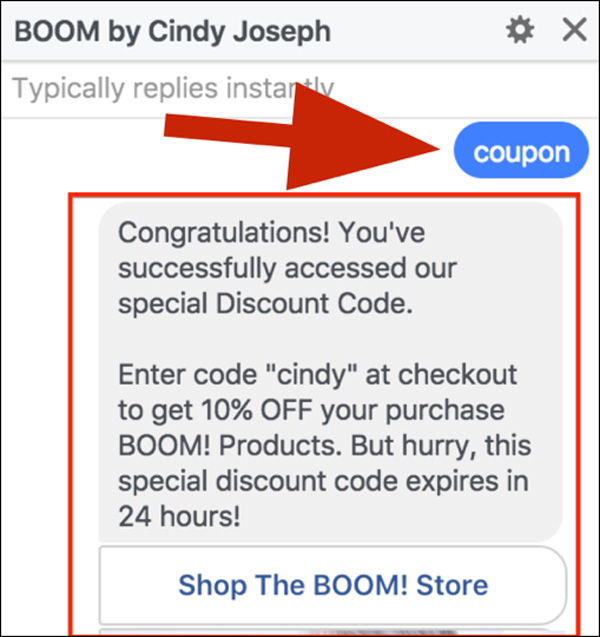The image depicts a close-up view of a promotional webpage containing multiple textual and graphic elements within a bordered box. The border is marked by a thin black line that encircles the content. 

At the top, there is a light gray line featuring a bold, capitalized rectangular bar that reads "BOOM by Cindy Joseph," flanked by a small gear icon on the left and an X on the right. Immediately below, on a white line, is the text "typically replies instantly."

Prominently in the center is a large red arrow pointing towards a blue oblong shape with "COUPON" written in white, uppercase letters. 

Further down, a red rectangle outlines a gray informational section that reads: "Congratulations! You've successfully accessed our special discount code. Enter code CINDY at checkout to get 10% off your BOOM products, but hurry, this special discount code expires in 24 hours."

At the bottom is another oblong shape, this time white with a gray outline, containing the text "Shop the BOOM! Store" in darker blue letters. Some content is partially visible below this section but is cut off and indiscernible.